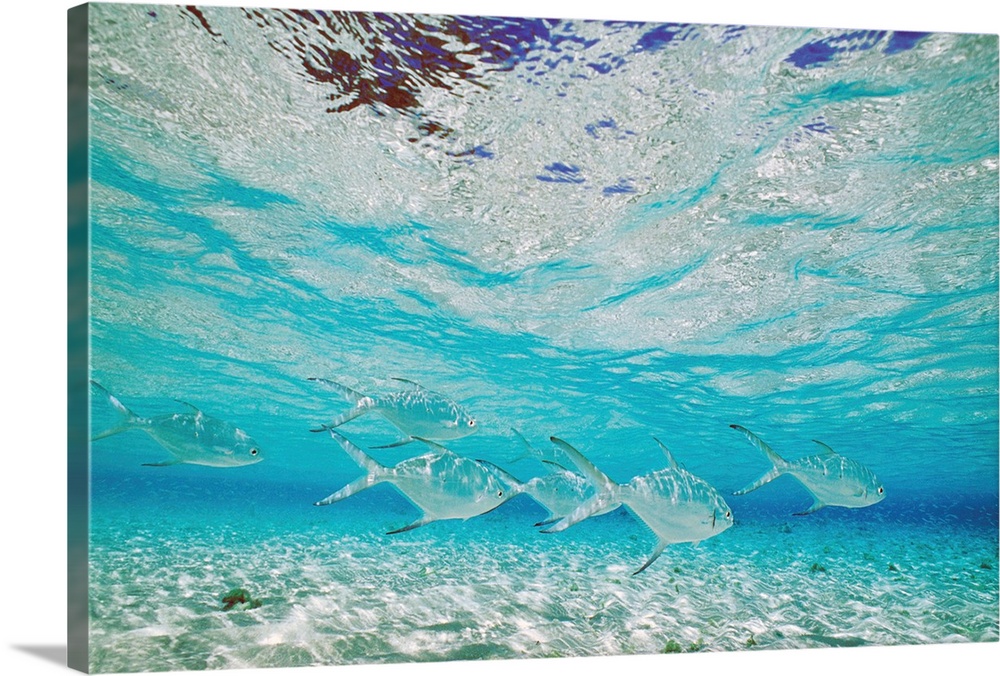The image is a serene and detailed underwater scene that is likely a high-quality photograph, though it has the appearance of being mounted on a canvas. The rectangular picture, oriented horizontally, captures a clear and pure aquatic environment, characterized by turquoise and greenish-blue waters. The surface of the water is slightly wavy, allowing glimpses of blue skies above. In the middle of the scene swims a school of six almost translucent fish, possibly tuna given their torpedo-shaped bodies, black beady eyes, and forked tail fins. These fish uniformly swim from left to right toward the edge of the frame. Below them, the seabed is visible, featuring clean sand and faint undergrowth, adding to the picturesque and calming atmosphere of the scene.